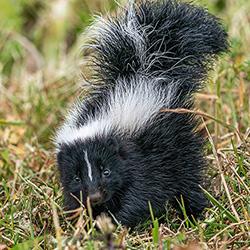This vibrant color photograph captures a curious and apprehensive baby skunk facing the viewer. The young skunk, characterized by its mostly black fur with distinct white accents, features two prominent white stripes running down its back and a thin white stripe across its forehead and nose. Its long, raggedy tail is upraised, though not in a spraying position. The skunk's fur is notably straight on its body and appears more disheveled on its tail. It stands amidst a patch of mixed green and brown grass, seemingly in a state of cautious curiosity. The natural setting is devoid of any humans, other animals, or structures, emphasizing the skunk's vulnerable position in the open grassy area. The skunk's tiny, beady black eyes give it an innocent yet wary expression as it appears almost reluctant to be photographed.